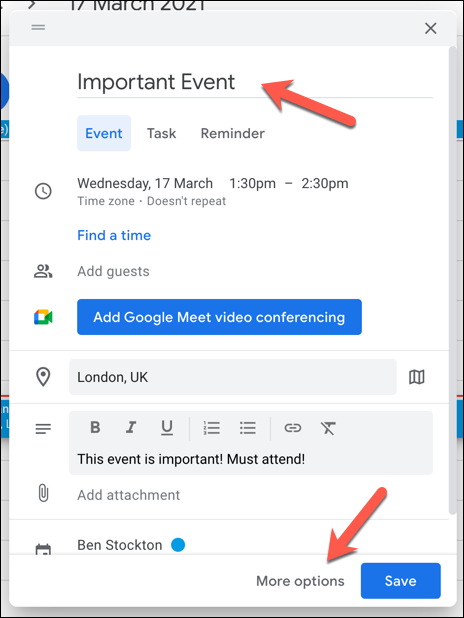A cropped screenshot showcases a website pop-up with a thin black frame and sharp corners. The pop-up itself is a white vertical rectangle with rounded edges, casting a medium gray shadow on the darkened white page behind it. The header of the pop-up is light gray, featuring a dark gray hamburger menu composed of two medium gray horizontal lines on the left, and a dark gray "X" on the far right.

In the body of the pop-up, large black text at the top left reads "Important Event." Below this text is a thin light gray line representing a text entry box. The following content includes three words: the first one, "Event," is in blue and highlighted within a light blue rectangle. To its right is the dark gray text "Task Reminder."

Further down, on the left side, a dark gray clock icon is present. Justified to the right of the clock icon are two lines of text. The first line is larger, in dark gray, and reads "Wednesday, 17 March, 1:30 PM-2:30 PM." Below this, left-justified light gray text reads "Time Zone," followed by a dot and the phrase "Doesn't repeat." 

Below the time details, slightly larger blue text reads "Find a Time," justified to the left. Underneath this, in quite small light gray text, the words "Add Guests" are displayed. To the left of this text, there is a dark gray icon depicting two people.